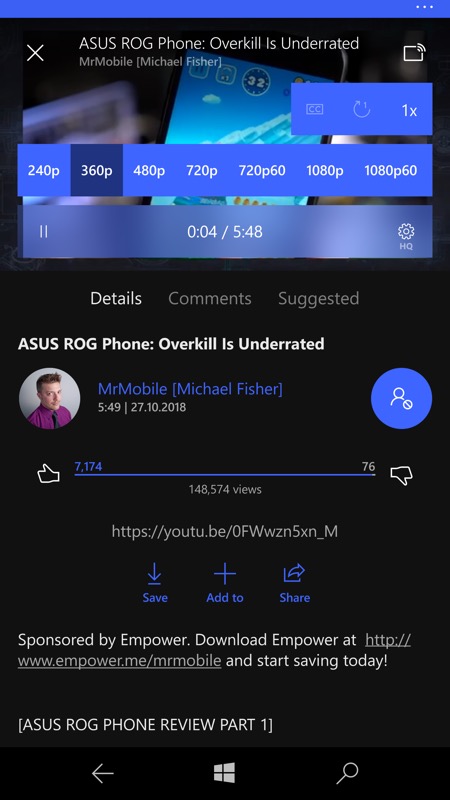The image shows a screen capture of a mobile application with a predominantly black background. At the top, there's a distinct purplish-blue border, followed by a title that reads "ASUS ROG Phone: Overkill is Underrated." Below the title is another purplish-blue bar displaying "1X," presumably indicating the playback speed. This is followed by another bar of the same color featuring video resolution options: 240p, 360p, 480p, 720p, 720p60, 1080p, and 1080p60.

The main section of the screen appears to be playing a video, indicated by a translucent purple overlay and a still image beneath it. The previous bars likely correspond to playback controls and video resolution settings. Below the video is a black section with white text displaying options for "Details," "Comments," and "Suggested," all centered for clarity.

On the left side, there's a photo of a user named 'Mr. Mobile'—real name Michael Fisher—suggesting he is either the reviewer or the person watching the video. Further down, users are provided options to give the video a thumbs up or thumbs down. At the very bottom, text reads "ASUS ROG Phone Review Part 1," noting that the review is sponsored by Empower, with an invitation to visit Gibb’s website for more information. Additional controls for navigating forward, searching, and the Microsoft logo are also visible.